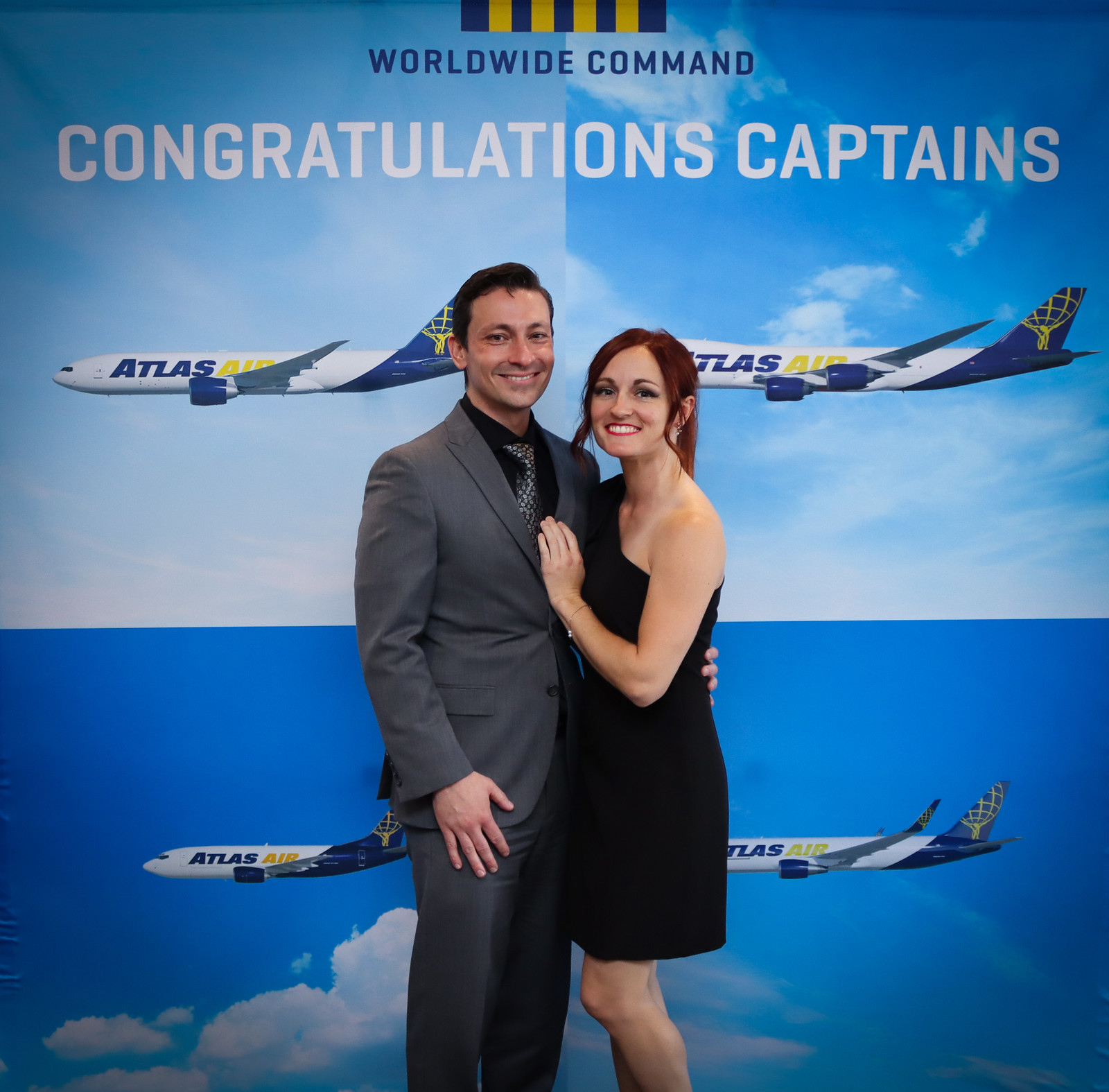In the image, a man and a woman are embracing and smiling at the camera. The woman is dressed in a short black, one-armed cocktail dress, exposing one arm and shoulder while the other is covered. She has red hair and is wearing red lipstick, with her hand resting gently on the man's chest. The man, standing to her left, is in a charcoal gray suit paired with a black dress shirt and a shiny black and silver tie. He has black hair and his arm is around the woman’s waist. Behind them is a backdrop featuring a poster that reads "Worldwide Command, Congratulations Captains," accompanied by four identical blue and white airplanes bearing the Atlas Air logo in blue and yellow. The celebratory setting suggests that the man may have recently graduated from commercial flight school.